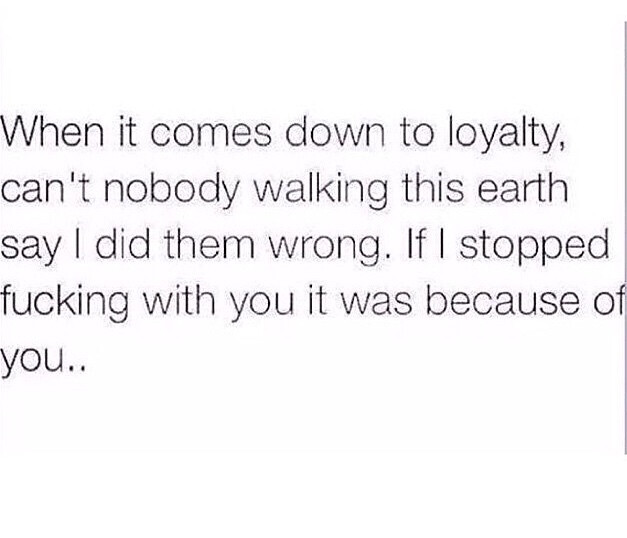The image features black sans-serif text, likely thin Helvetica, centered against a white background. The text appears slightly pixelated in the middle, indicating lower image quality, perhaps from a screenshot. The content reads: "When it comes down to loyalty, can't nobody walking this earth say I did them wrong? If I stopped fucking with you, it was because of you..." A single black line is present on the right-hand side, with no additional imagery or attribution for the quote.